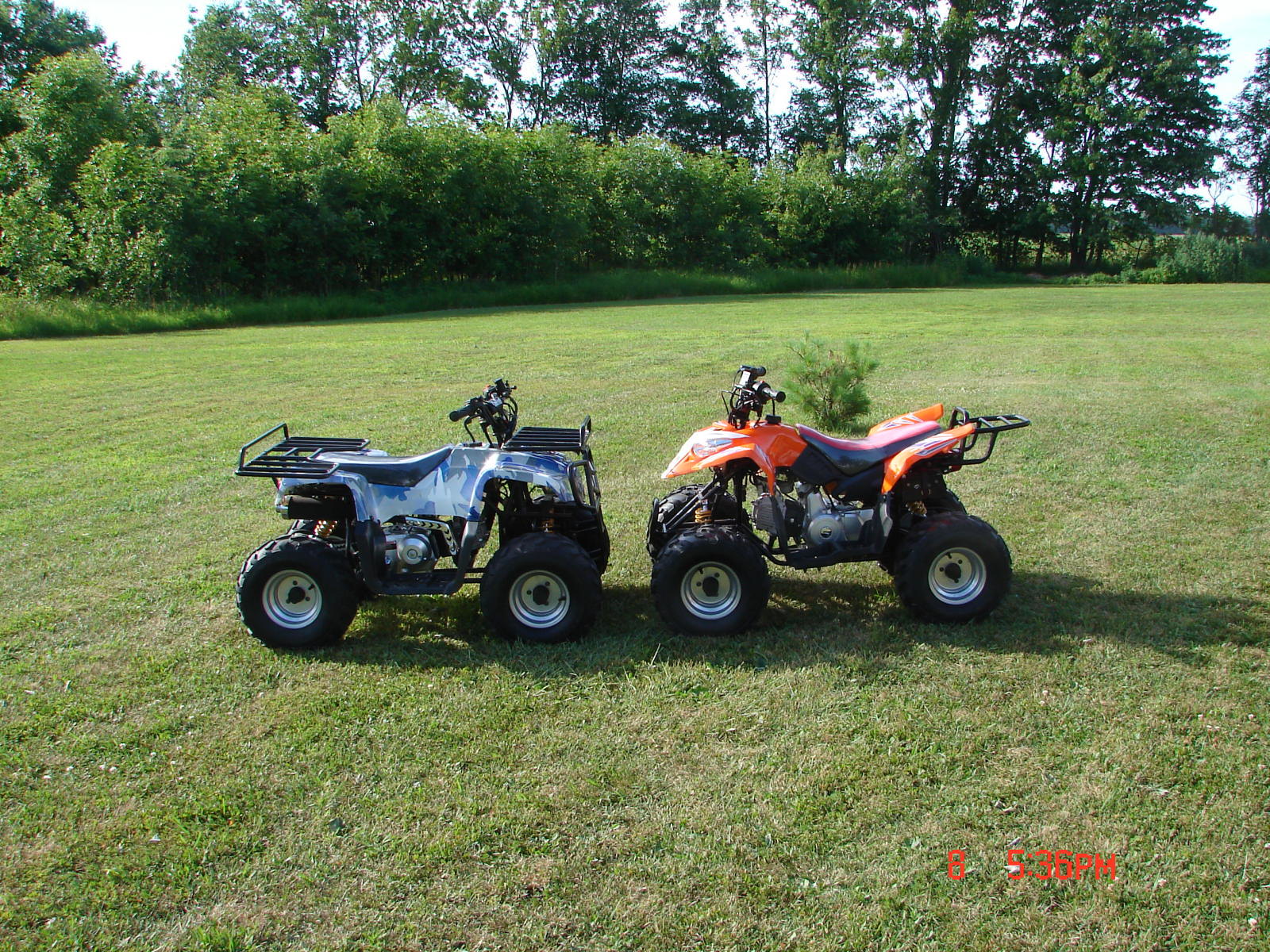In this outdoor photo, two children's ATVs are parked facing each other in a field of green grass. The ATV on the left features a boxy design, a blue camo finish, a black seat, and a front rack. In contrast, the ATV on the right has a more rounded and angular design, is primarily orange-red with a red seat, and has a rear rack. Both vehicles seem to be of similar models, sharing components like motors and wheels, which are largely identical. Behind the red-orange ATV, there is a small shrub or tree. In the background, a mix of tall, green and bushy trees become visible, gradually transitioning to a more densely forested area with additional trees and possibly mountains in the distance. The clear sky and the shadows cast by the ATVs hint at good weather, with the time stamp "5:36 p.m." in red lettering appearing at the bottom right corner of the image.